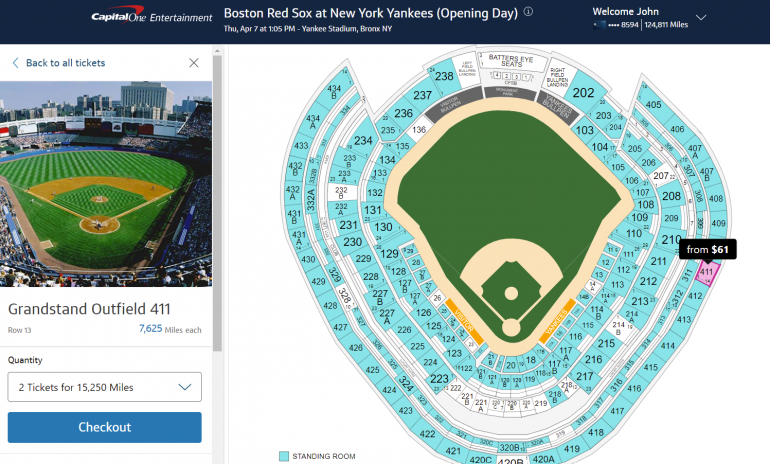This detailed screenshot in landscape mode, likely taken from a laptop, features Capital One Entertainment's web interface. The top portion of the image has a dark blue background, with the Capital One logo prominently displayed to the left and the word "Entertainment" in italics. 

Just below, the event details are shown: "Boston Red Sox at New York Yankees (Opening Day)". An information icon, represented by an eye in a circle, is positioned nearby. The specifics of the event are listed: "Thursday, April 7th at 1:05 p.m. Yankee Stadium, Bronx, New York". On the upper right corner of the screenshot, a greeting displays: "Welcome, John". Next to the greeting are figures "8594" and "124,811 miles", indicating the user's balance of Capital One miles.

The content is organized into two columns. The left column begins with a link labeled "Back to All Tickets", followed by an image depicting Yankee Stadium and an overlay showcasing the seat view from "Grandstand Outfield 411". The cost for these tickets is listed as "7,625 miles" each, with an option to purchase two tickets for a total of "15,250 miles" and a blue "Checkout" button below.

The right column features detailed ticketing information. A display section for Yankee Stadium is shown, with a pink button at the far right stating "From $61". The seat section "411" is highlighted in pink, marking it clearly.